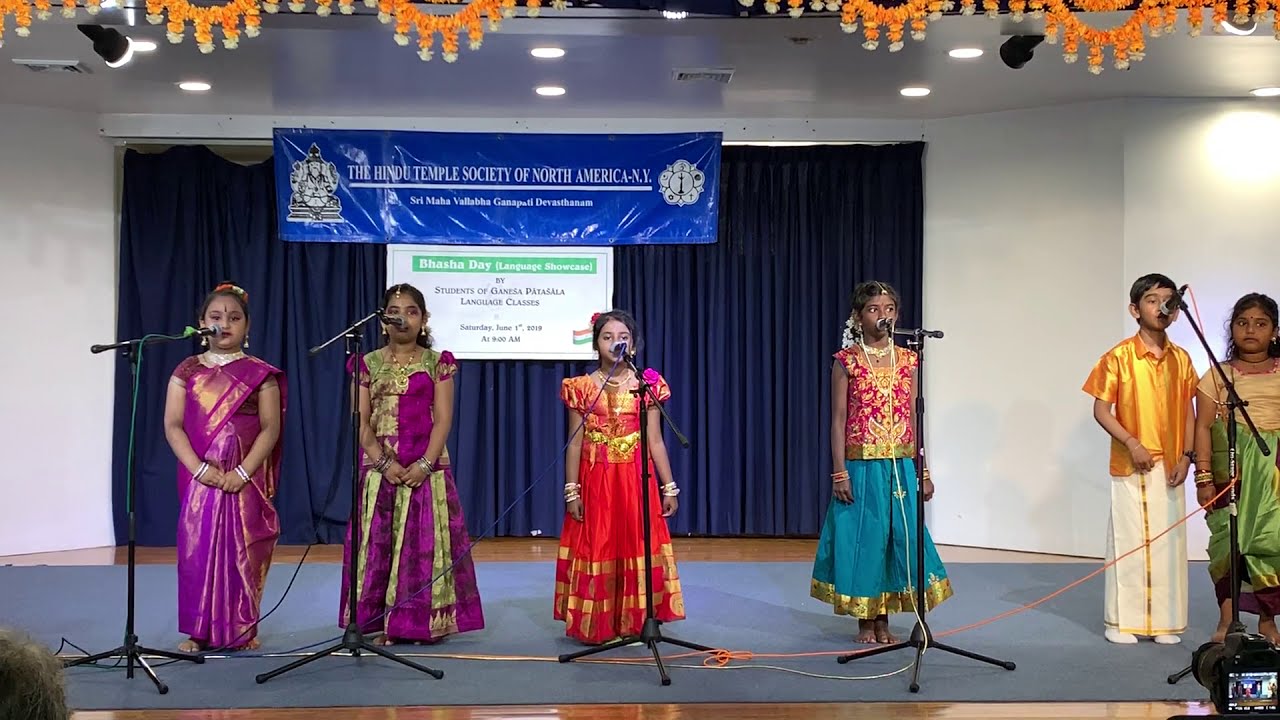On a stage adorned with blue curtains and festive gold-and-white decorations, six children stand lined up, performing at a microphone each. The event is hosted by the Hindu Temple Society of North America, New York, with a visible banner and a white sign detailing the occasion. The children are garbed in traditional Indian dresses of varying but coordinated colors. On the far left, a girl in a dark purple dress with a ponytail peeks out, only her sleeve visible. Next to her stands another girl in a purple dress with golden-green stripes accentuating the shoulders, chest, and hem. Center stage, under a prominent light, the shortest girl in a red dress with golden embellishments and matching wristbands captures attention. To her right is the tallest girl, combining a red top with a blue skirt trimmed in gold, offset by reddish-white bracelets. Sharing a microphone on the far right, a boy in a golden shirt and white pants sings, flanked by a girl in a tan top and green skirt. The stage floor consists of a gray rug over wooden flooring, and the supportive audience can feel the cultural richness and unity conveyed by the children’s performance.